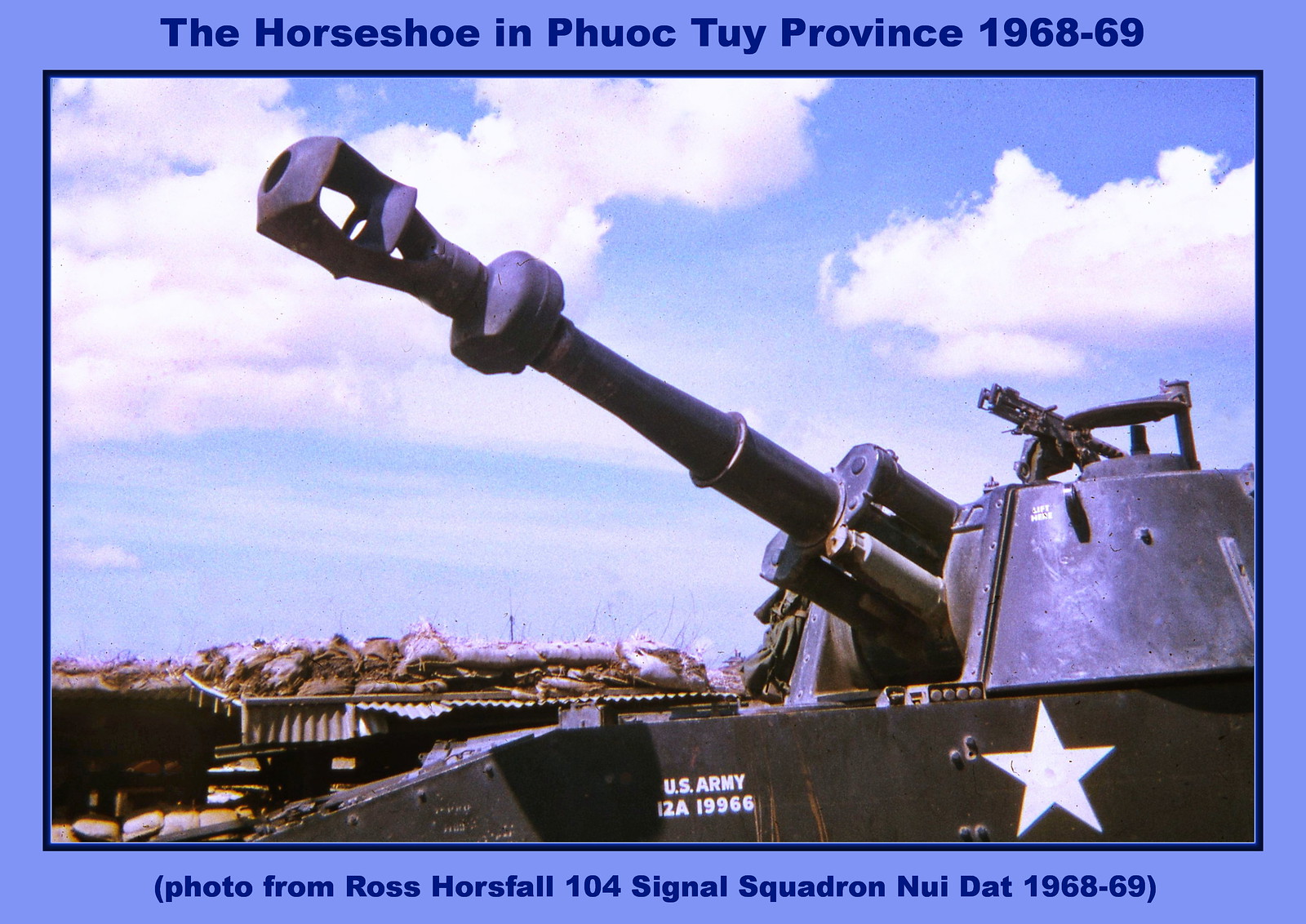This detailed photograph captures a U.S. Army tank in a historical setting from 1968-69. The image is accented by a black border and features a light blue background with scattered clouds. Dominating the foreground is the tank, clad in dark gray and black, with its gun barrel angled to the left. Adorning the side of the tank is a noticeable white star and the identifier "U.S. Army 12A-19966" in crisp white letters. Above the photo, in dark blue font, the text reads, "The Horseshoe in Phuoc Toi Province 1968-69," while the bottom of the image contains the credit, also in dark blue, "Photo from Ross Horsefall 104 Signal Squadron Nui Dat 1968-69." In the background, piles of what appear to be sandbags or debris are visible, hinting at the rugged environment.